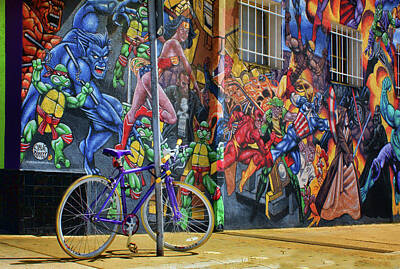This small, rectangular image captures a vibrant, bustling street scene dominated by a bicycle securely chained to a metal pole positioned slightly left of center. The setting suggests a sidewalk adorned with a rich brownish floor that resembles either dirt or wooden planks. Behind this bicycle, a vividly painted mural adorns the wall of a building, creating a striking and colorful backdrop. This elaborate mural features an array of comic book and superhero figures, including recognizable characters such as the Ninja Turtles, the blue guy from X-Men (likely Beast), Captain America, and what appears to be the Flash. The mural showcases an energetic display of characters in bold and vivid colors, with some figures wielding weapons like swords and nunchucks, and others captured in dynamic action poses. The upper right section of the wall features a balcony with additional painted figures, contributing to the rich tapestry of this colorful scene. The street setting, with its detailed mural, colorful superhero ensemble, and urban elements like the metal pole and sidewalk, collectively creates a lively and eye-catching image.